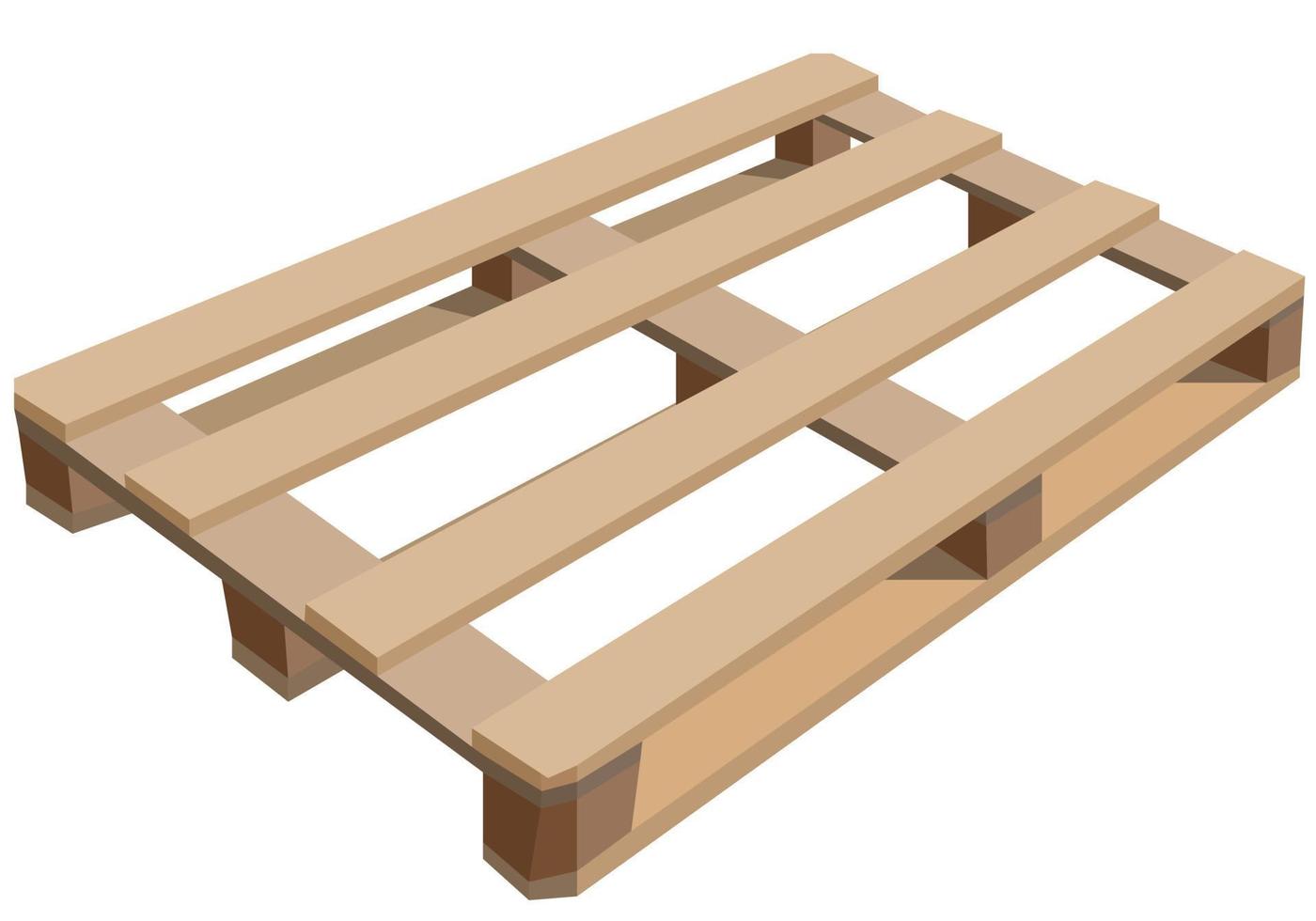The image depicts a light tan, digitally rendered, low-poly wooden pallet set against a completely white background. The pallet consists of four horizontal slats on top, with three perpendicular slats directly underneath, and an additional three slats forming the base. The angle of the image positions the viewer as if standing at a corner of the pallet, about two feet away and looking down diagonally. The overall design appears smooth and modern, resembling computer-generated imagery, and while it might not be functional for holding items, it serves well as a platform for elevating objects off the ground. The pallet’s simplistic and clean design allows for versatile uses, such as stacking multiple units to create a broader storage surface.